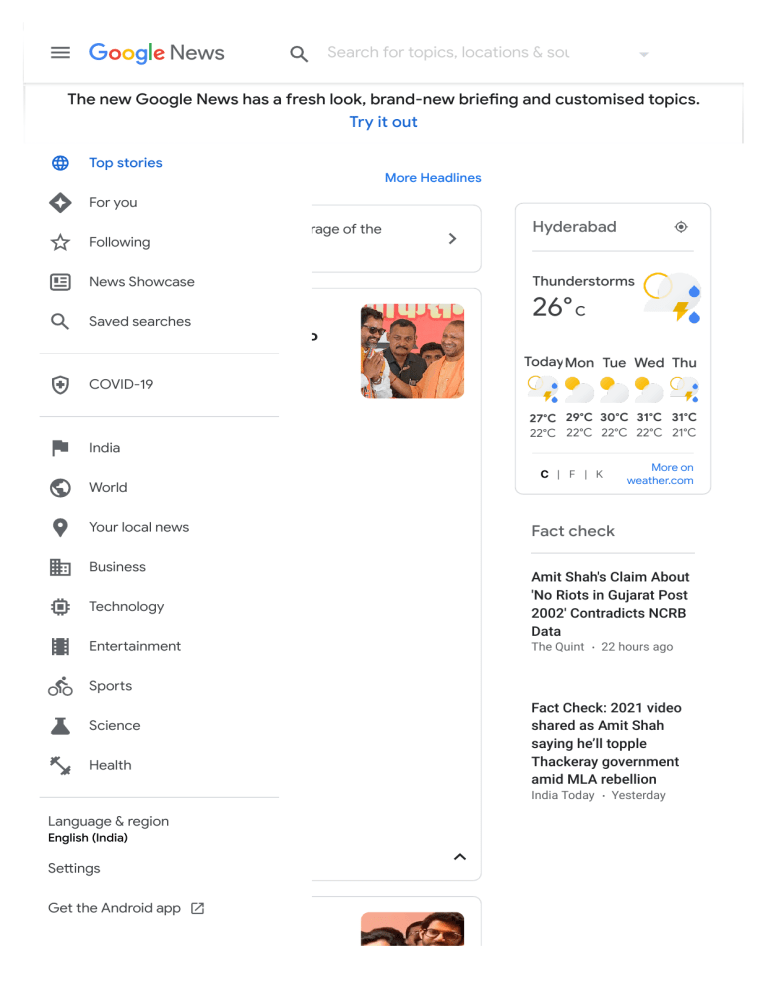This image is a screenshot of the Google News interface in portrait mode. 

In the upper left-hand corner, there are three horizontal gray lines indicating the menu icon. Next to it, the text "Google News" is displayed, followed by a search icon. The search bar contains the placeholder text, “Search for topics, locations, and...” but it's in a very faint gray that's difficult to discern against the white background.

Directly below this, a gray horizontal line separates the search section from the main content. In bold black text, it reads, “The new Google News has a fresh look. Brand new briefing and customized topics.” Followed by the prompt "Try it out" in blue text, which is a clickable link.

On the left column, the menu options are listed:  
- Top stories (highlighted in blue)
- For you
- Following
- News showcase
- Saved searches
- COVID-19
- India
- World
- Your local news
- Business
- Technology
- Entertainment
- Sports
- Science
- Health

There's another gray line breaking this section which ends with "Language and region is English (India)," alongside options for "Settings" and "Get the Android app."

In the upper center of the interface, directly beneath the "Try it out" link, there's a segmented heading for "More headlines" in blue text, a clickable link.

On the right side of the screen, weather details for "HYDERABAD" are displayed. It shows thunderstorm icons with the current temperature at 26 degrees Celsius. The forecast for today through Thursday shows temperatures ranging from 27 to 31 degrees Celsius. Below this, a link to “More on weather.com” is provided in blue text.

In the content section below the weather, there’s a fact-checked article stating: “Amit Shah's claim about no riots in Gujarat post-2002 contradicts NCRB data.”